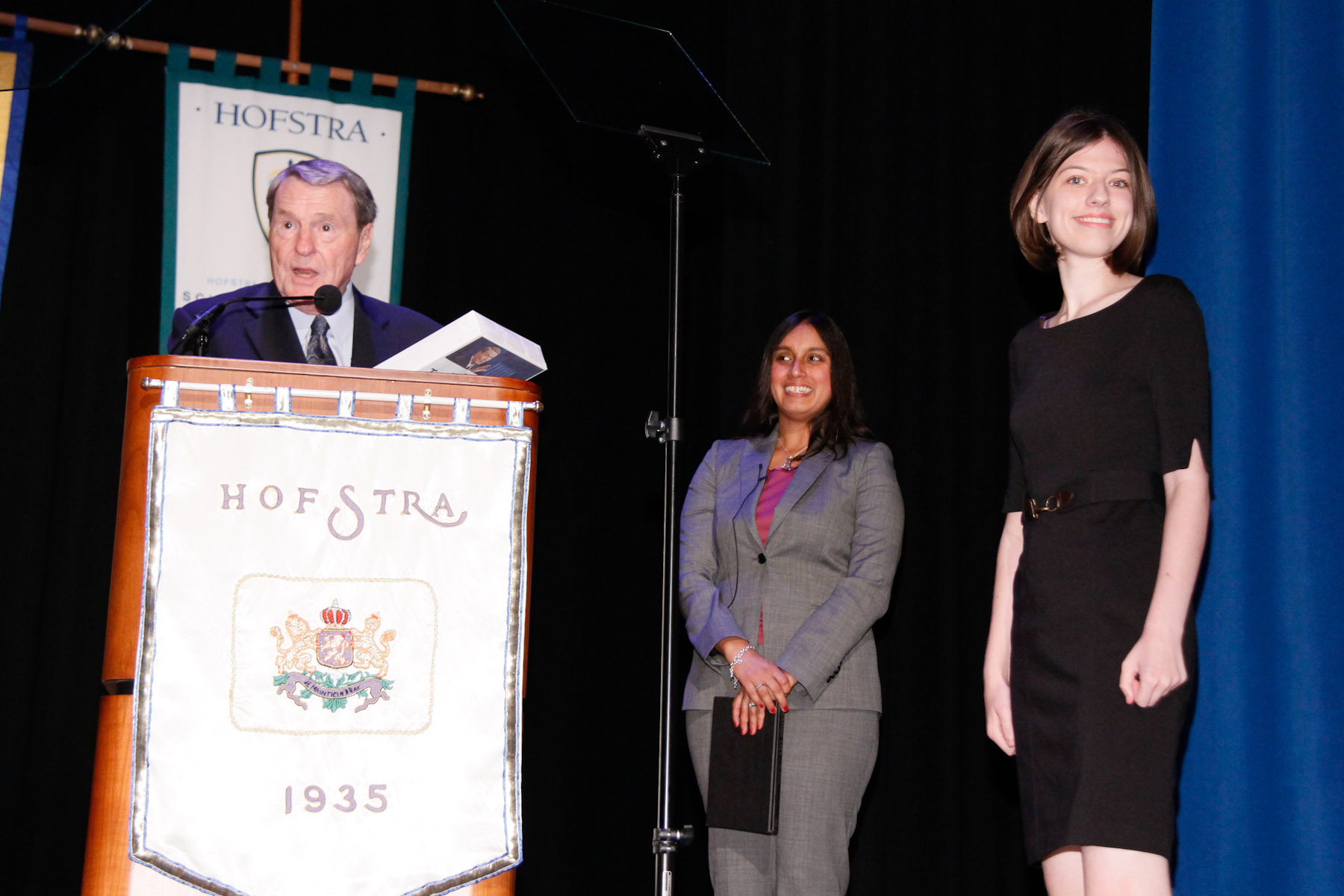In this photograph, three people are standing on a stage with a black curtain and a blue curtain in front of it. At the center is a man with short gray hair, dressed in a dark blue suit with a white shirt and a dark blue tie. He is speaking into a microphone from behind a large podium that bears a banner with the name "Hofstra" and the emblem of the university, along with the year 1935. Beside him stands a tall pole with a teleprompter perched high above, resembling a tall music stand.

To the right of the man, there are two women. The woman closest to the man is an Indian woman with long brown hair, dressed in a gray business suit paired with a pink shirt, and holding a black notebook in her hands. The second woman, standing to the far right of the photo, has medium-length straight brown hair styled in a bob. She is wearing a professional black dress with a small belt and is smiling warmly at the camera. Both women are positioned slightly to the front, with the podium and the man behind it as the central focal point of the image. The backdrop includes a green and white tapestry further emphasizing the "Hofstra" theme.